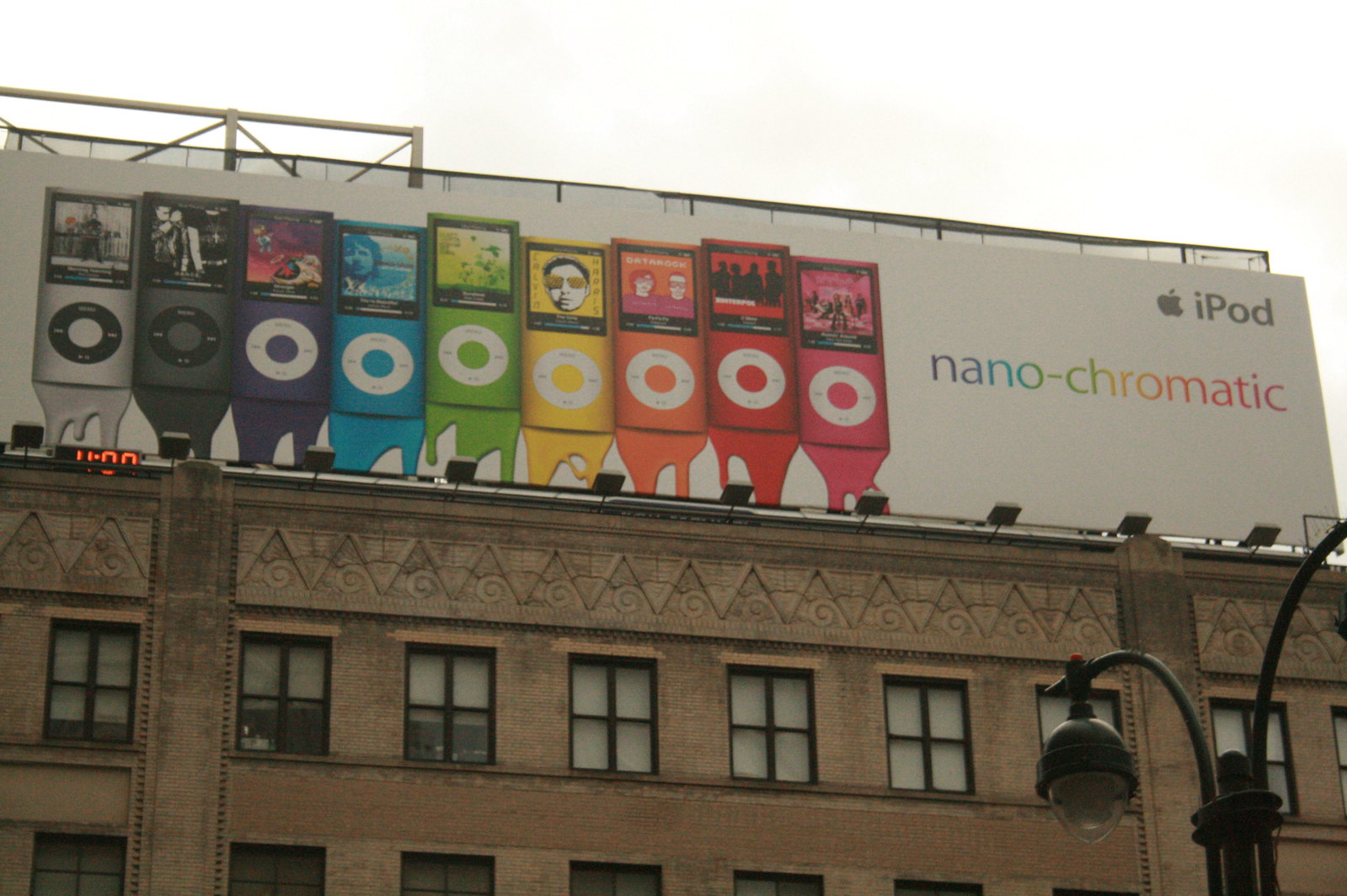The image features a striking billboard affixed to the facade of a gray cement building lined with several black-framed windows. The billboard itself is white and prominently displays a series of colorful iPods arranged from left to right: gray, black, purple, turquoise, lime green, yellow, orange, red, and pink. Above the vibrant lineup of iPods, in the upper right-hand corner, the iconic Apple logo and the word "iPod" are positioned, with the term "nanochromatic" featured prominently to the right of the devices. The base of the building is illuminated by track lighting, casting a subtle glow on the structure. In the foreground, there is an older-style black wrought iron street light, adding a touch of vintage charm to the scene.